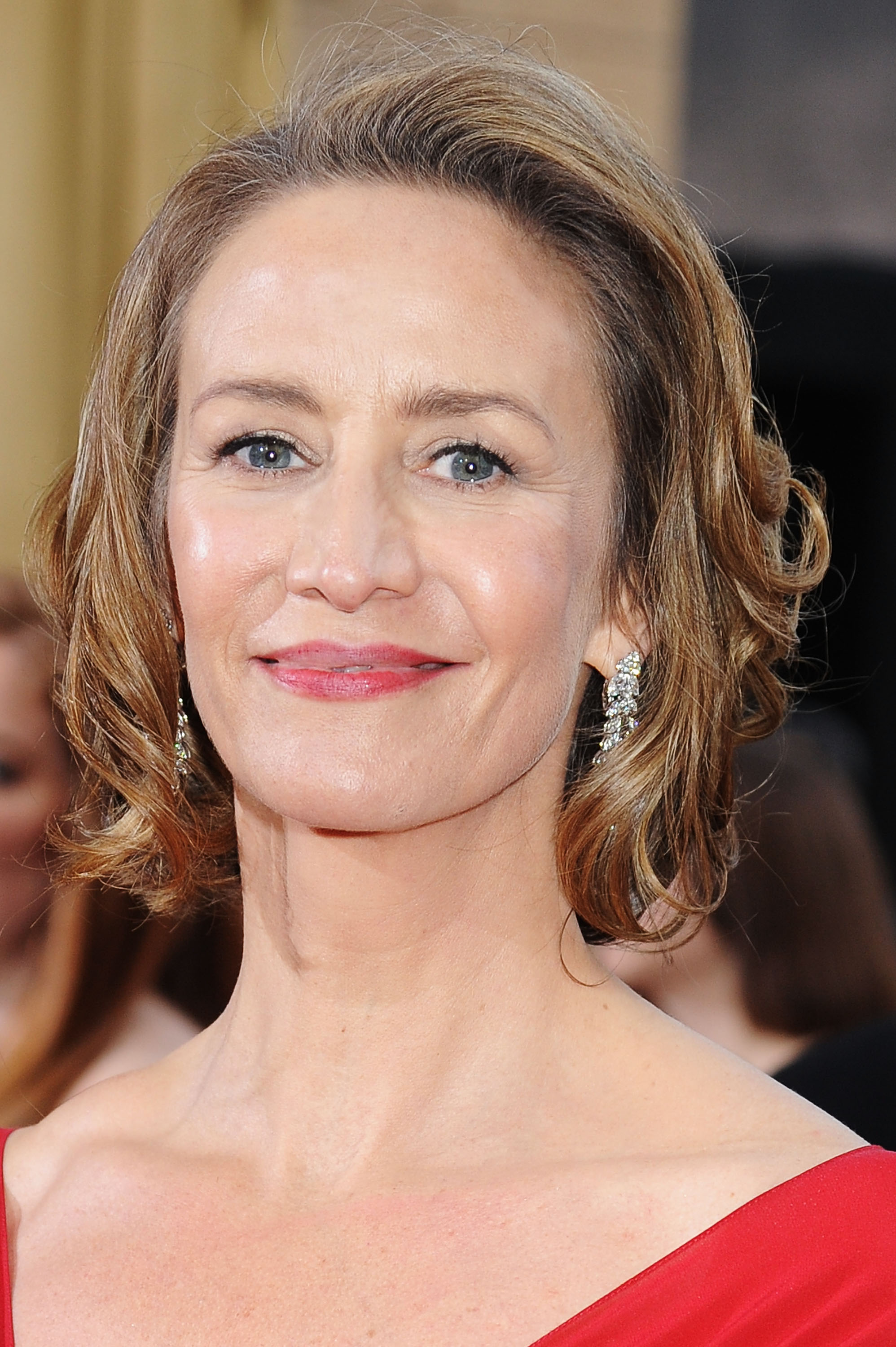This close-up photograph captures a detailed image of an older white woman, possibly an actress attending a red carpet event or movie premiere. Her light brown hair, slightly graying at the top, falls just below her jawline. She has striking bluish-gray eyes and wears red lipstick, which complements her gentle, closed-mouth smile. Her red dress is partially visible at the edges of the rectangular photo, and she is adorned with large diamond earrings. Though the background is blurred, it suggests the presence of other attendees, enhancing the atmosphere of the glamorous event.